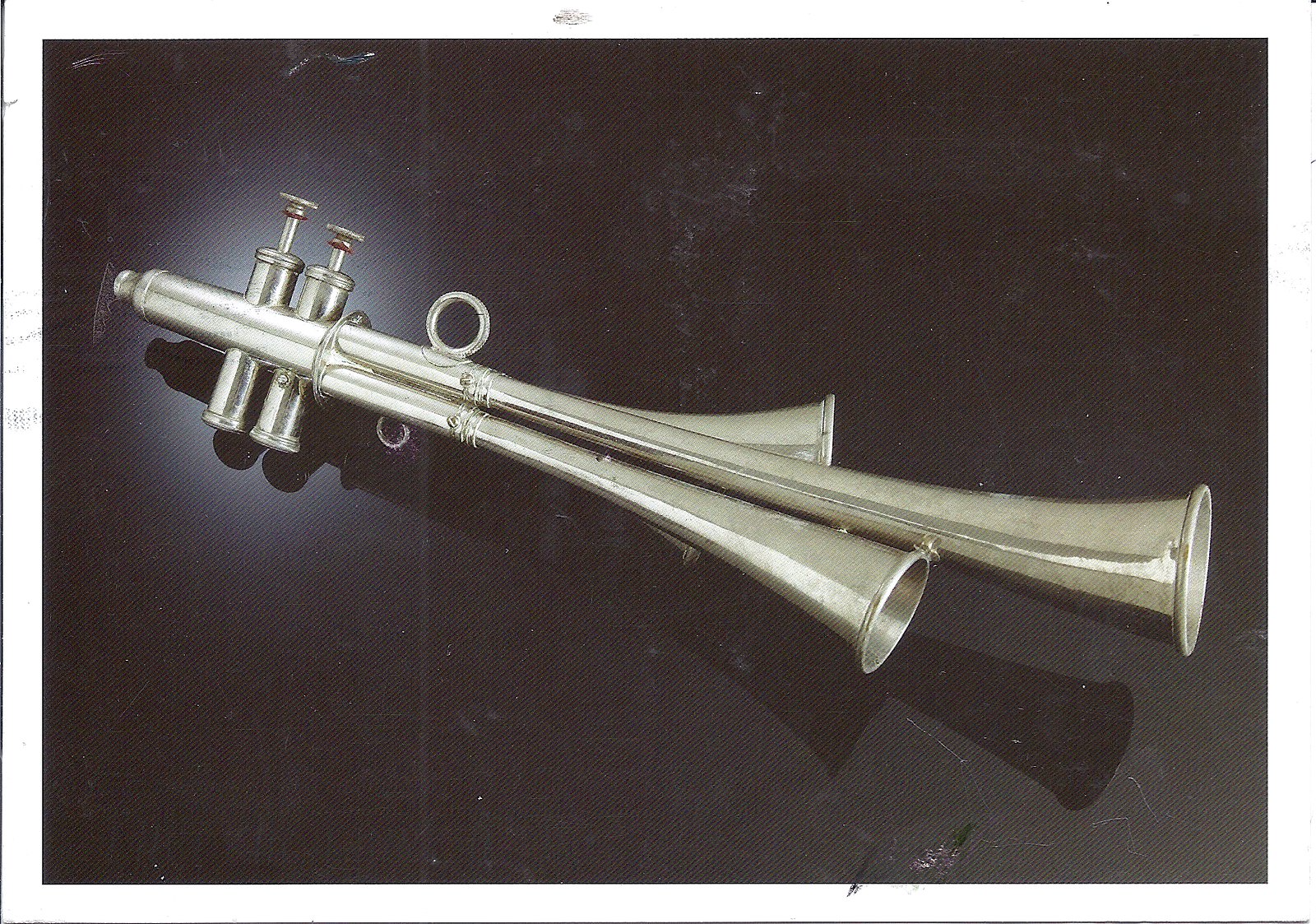The image depicts a silver-colored brass musical instrument, resembling a hybrid of three trumpets merged into one. It features three distinct horns at the bottom: the central horn is the longest and curves upwards, while the other two are shorter with one straight and the other curving away. All three horns converge into a single mouthpiece. The instrument is adorned with two large pronged valves on the left side, facilitating sound modulation. Additionally, there are circular finger rings at the top and bottom for handling. The instrument is centrally positioned against a black background with varying shades, darker in the upper left-hand corner and lighter towards the lower right-hand corner, giving the backdrop a scratched or ripped paper appearance. The lighting accentuates the instrument's reflective silver surface, highlighting its unique structure and intricate details.